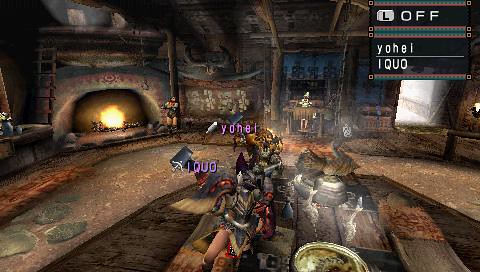This detailed screenshot from the video game "Monster Hunter" showcases an online hub where players have gathered. In the scene, several characters are outfitted in elaborate medieval sci-fi armor, suggesting they are prepared for battle. Prominent names like "Y-O-H-E-I" and "I-Q-U-O" are displayed, likely identifying these characters as players in the game. The setting features a large, blazing stone fireplace, surrounded by a pile of firewood, adding a rustic ambiance to the rugged dirt and rock floor. An entryway is visible on the right, enhancing the immersive environment. In the top right-hand corner, game indicators are visible, with text reading "L off," providing game status updates.